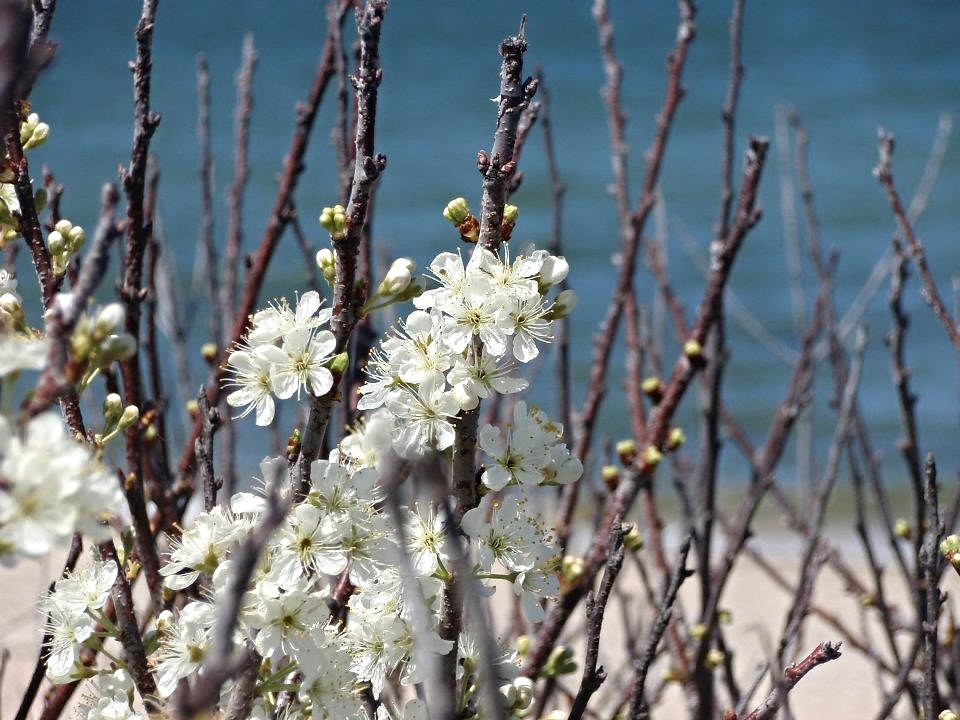This detailed, close-up photograph captures the serene beauty of cherry blossoms just beginning to bloom in the spring. The central focus is on the crisp, white petals with a mixture of cream hues, dotted with patches of lemon green, creating a calm and delicate appearance. Several clusters of blooms and buds are prominently displayed, some still tightly closed while others have fully opened, revealing green or yellow centers. The thick stems and branches support these delicate flowers, with some showing signs of withering in the background. The outdoor setting suggests a beach, with a hint of calm blue water in the blurred backdrop, giving the image a tranquil, natural ambiance. The entire composition is artistically framed, bringing out the contrast between the sharp floral details and the soft, blurry background, hinting at an overcast sky with patches of dark blue and grey.